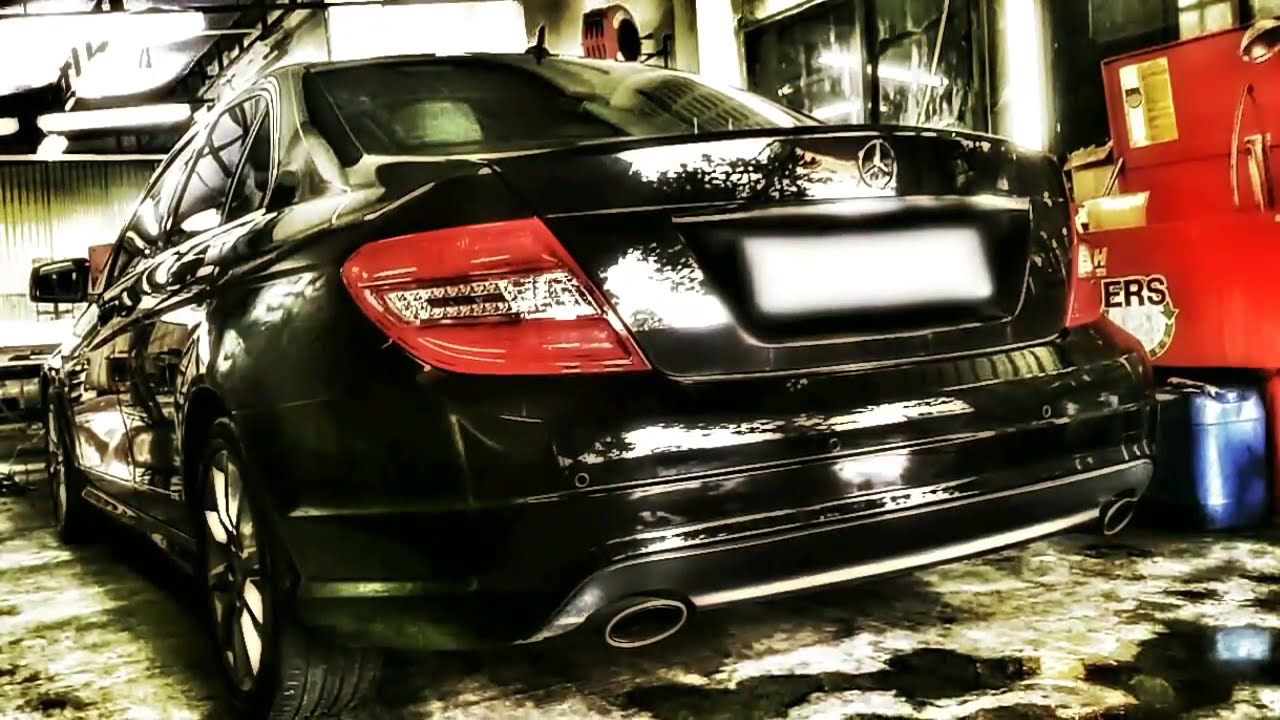The image portrays an edited photo of a sleek black car, likely a Mercedes-Benz, captured from a low angle at the rear, emphasizing its left taillight. The car’s glossy finish reflects multiple light sources, making it appear almost in motion despite being parked inside a garage. The garage, looking somewhat industrial and processed, has a distinct red toolbox with an indistinct logo containing "ERS" on the bottom right. Overhead lights cast strong reflections on the vehicle and the gray-silver concrete floor, which exhibits patches suggestive of either a textured surface or liquid reflections. The ceiling and partial walls of the garage include window panes and corrugated metal, adding to the industrial ambiance. The image is heavily edited to enhance highlights, contributing to its partly black-and-white appearance, giving sections of the photo a blown-out look.